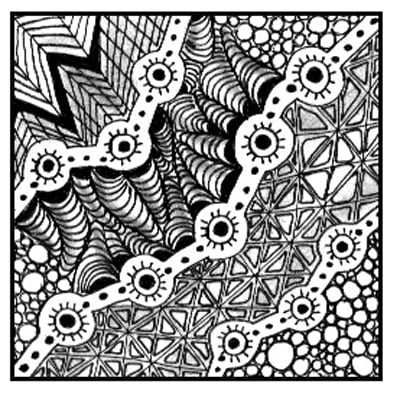The image depicts a highly detailed and intricate black-and-white drawing or print, formatted within a perfectly square frame bordered by a quarter-centimeter-thick black line. Each side of the square is of equal length, giving a balanced and symmetrical appearance. The drawing, executed with what appears to be charcoal or pencil, lacks any color, text, animals, or people, focusing solely on geometric shapes and abstract designs.

In the top left corner, a series of inward-pointing chevron patterns culminates at a black wavy line, which is intersected by a chain of equally spaced white circles connected by white rods featuring black dots inside, resembling eyes with "eyelash" details. Further to the right, the design evolves into a complex formation of stacked, conical shapes that resemble a three-dimensional effect, reminiscent of tiled peaks or striped rooftops.

Moving to the center of the artwork, a striking feature is the conical tubes emanating outwards, surrounded by the interconnected chain of circles with eyes, creating a dynamic focal point. This central pattern is bordered by more white lines with equally spaced eyes, adding layers of depth.

On the top right and bottom left quadrants, the artwork is populated with various round shapes of different sizes, often interconnected and creating a cohesive, yet varied, pebble-like texture. These sections are divided by additional white lines featuring the recurring eye motif, enhancing the theme of interconnectedness.

In the bottom right corner, the design transitions into a cluster of roundish forms that vary in size and are termed as 'pebbles,' juxtaposed with 'boxed X' patterns. These 'boxed X's' are squares containing an uppercase gray X, intersected by a smaller black X, all set within a light gray box border.

Overall, the image is an engaging and multifaceted composition of geometric patterns and abstract motifs, seamlessly blending cones, circles, and intersecting lines to create an intriguing and balanced visual experience.